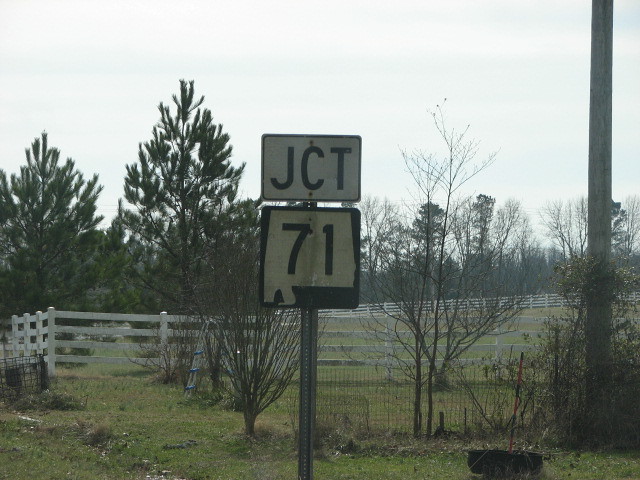The image features a road junction sign prominently displayed on the side of a rural roadway. The sign is structured into two distinct sections, both featuring a white background with black text. The top section is a rectangular sign with the abbreviation "JCT" in bold black letters, indicating a junction. Below it, the second section is a slightly weathered square-shaped sign with the number "71" also in black font.

The background reveals a pastoral setting, reminiscent of a farm. A white, horizontally-slatted picket fence runs parallel to the road, likely serving to contain livestock or mark property boundaries. The overall scene exudes a rustic charm, with the utilitarian road sign standing in contrast to the bucolic landscape.